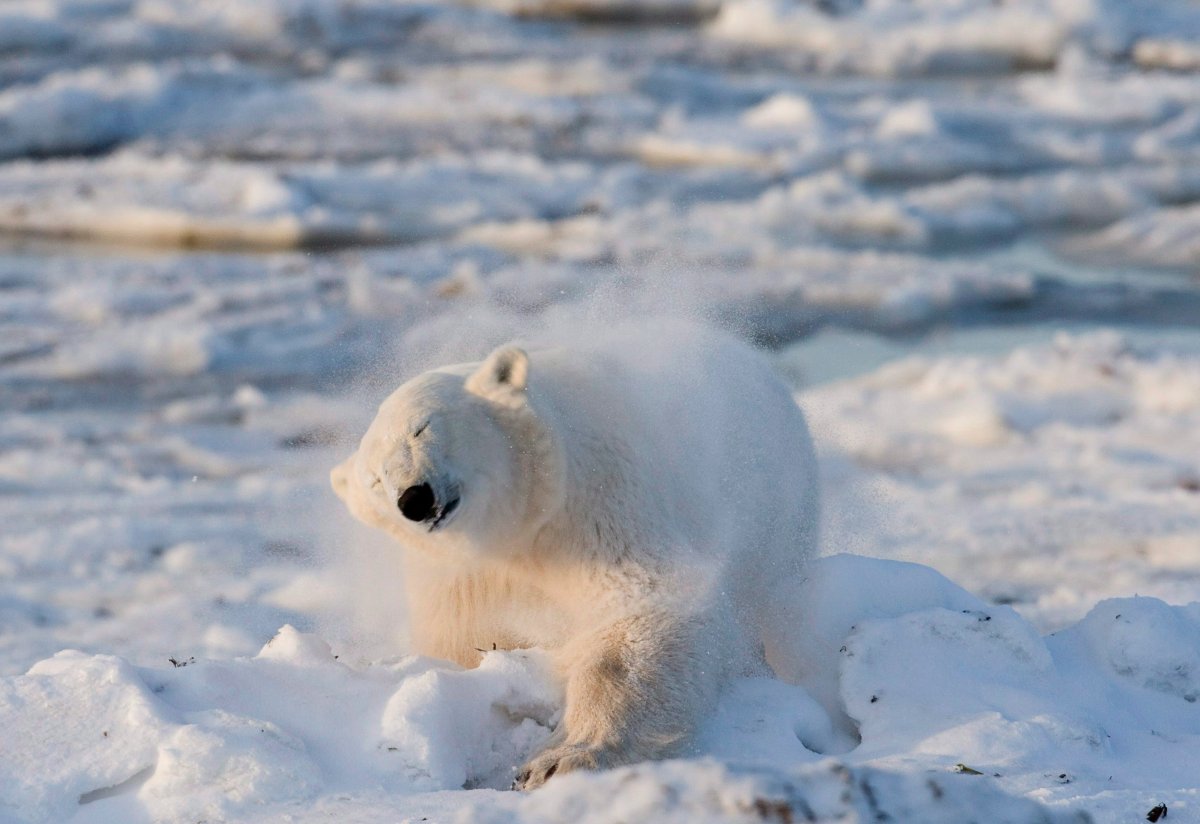The image captures a peaceful scene of a large, white polar bear navigating through deep snow. The bear, appearing content and calm with its eyes closed and head slightly tilted, is in the process of dusting off snow from its paws. The polar bear's massive, hulking presence is prominent, though its peaceful demeanor suggests a sense of tranquility. Surrounding the bear is a frigid landscape featuring sheets of ice on the water, reinforcing the cold environment. Despite its seemingly bulky size, the polar bear's herbivorous diet adds an intriguing layer to its majestic appearance.